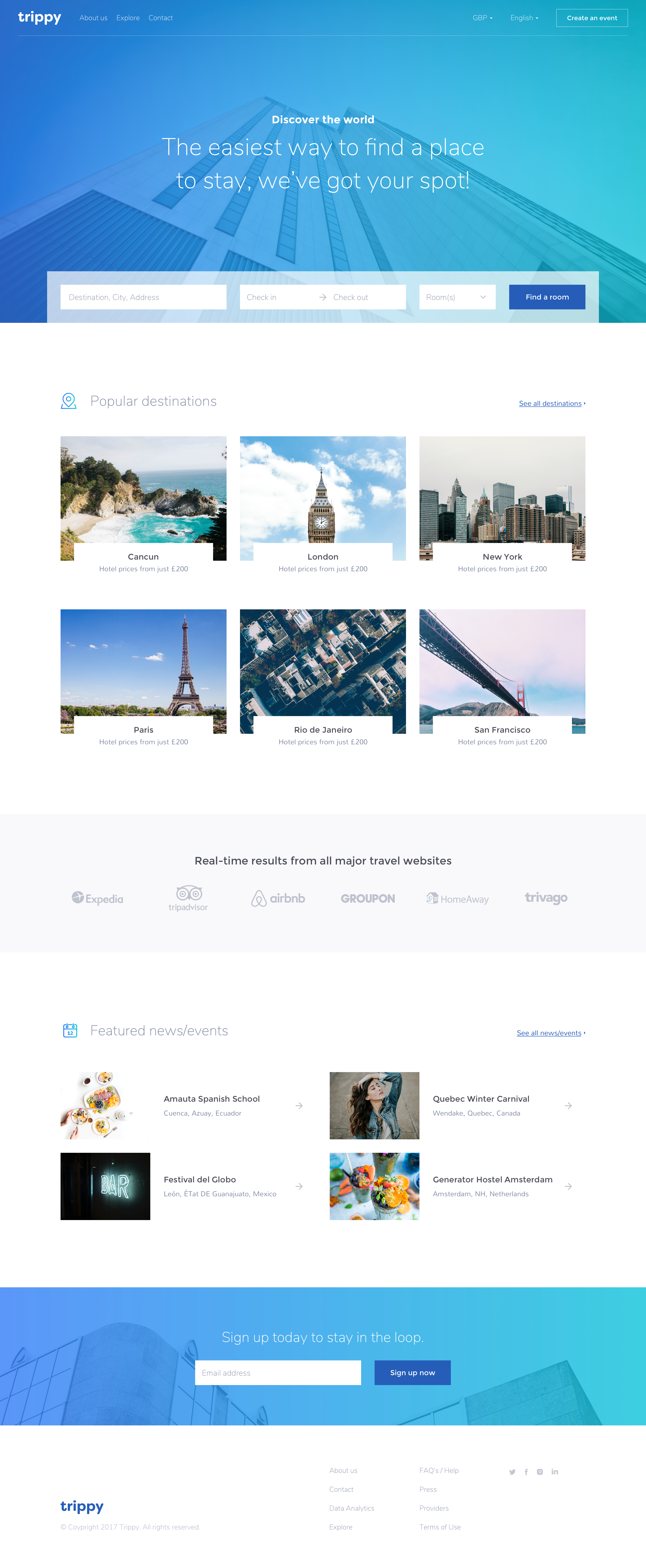The image features a primary blue box at the top, prominently displaying the word "Trippy" in white text. Surrounding this title is smaller, less legible white text on both its left and right sides. Centrally located on the image is a bold white print stating, "The easiest way to find a place to stay. We've got your spot." Below this, there are three white boxes within the blue box, accompanied by a blue button.

The background of the image is white, with additional small print at the very top, and a small blue box is also visible. On the right side, there are blue prints and six vibrant pictures showcasing mesmerizing places to stay, featuring stunning cityscapes and scenic views.

Further down, there’s another small blue box containing tiny blue text alongside a miniature blue icon, followed by more small blue print. Four more smaller pictures are arranged in this section, highlighting more beautiful locations.

At the bottom is a large blue box with white text, including a search box and an adjacent blue button. In the footer on a white background, the word "Trippy" reappears in blue text.